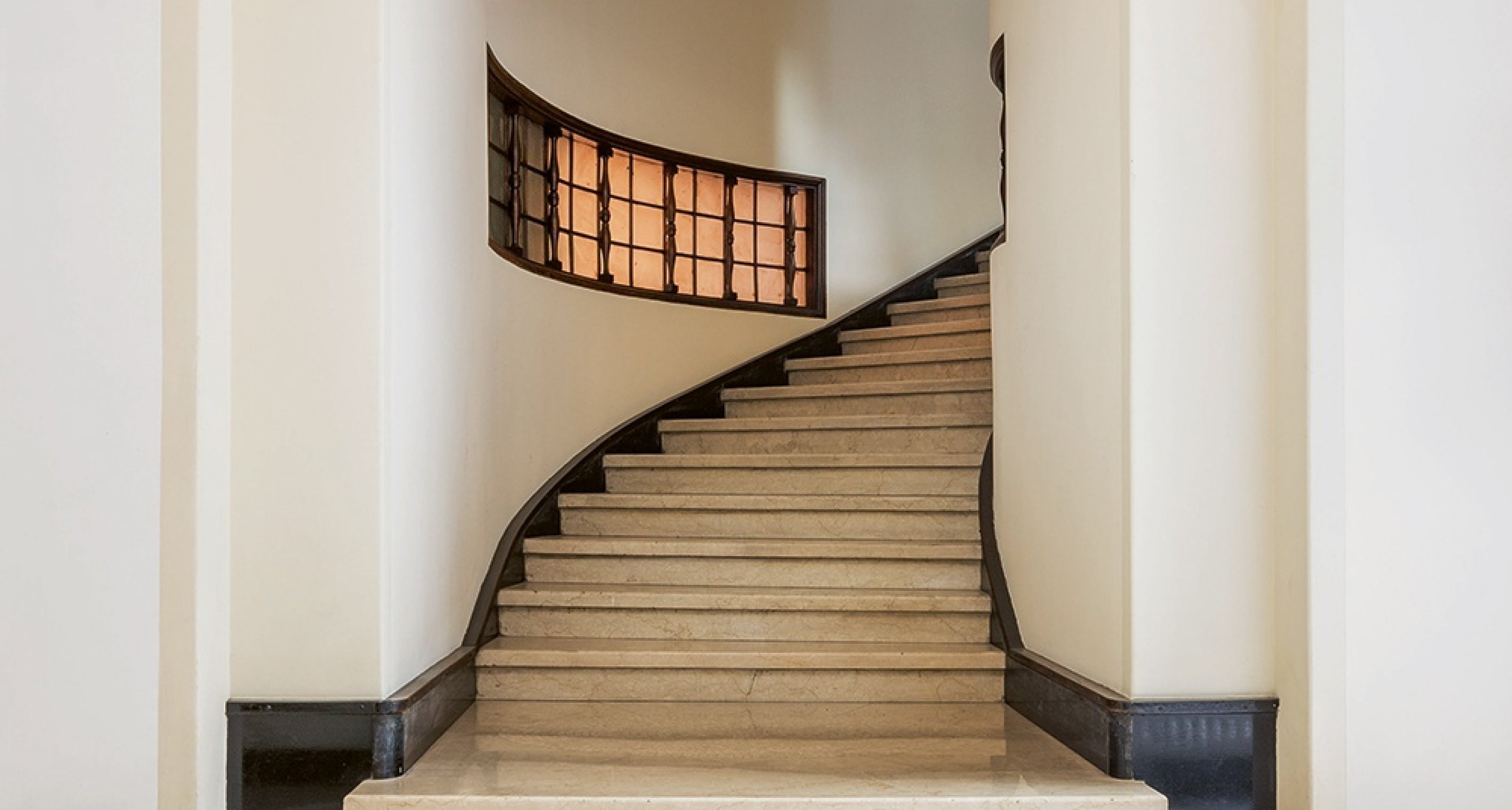This detailed photograph captures an elegant, winding staircase in a sophisticated indoor setting, possibly a fancy home or a mansion. The staircase, centrally positioned and leading upward while curving to the right, is constructed from beige marble, accented with dark brown or black baseboards. The structure exudes luxury and refinement. To the left of the staircase, a round window set against clean, white walls draws attention. This window, possibly made of colored or tinted glass, subtly illuminates the scene without revealing a clear view outside. The image's color palette includes various shades of white, off-white, beige, tan, and hints of black, creating a warm yet minimalist and pristine atmosphere. The photo itself has a wider aspect ratio, similar to that of a high-definition television screen, further emphasizing its artistic and serene composition.